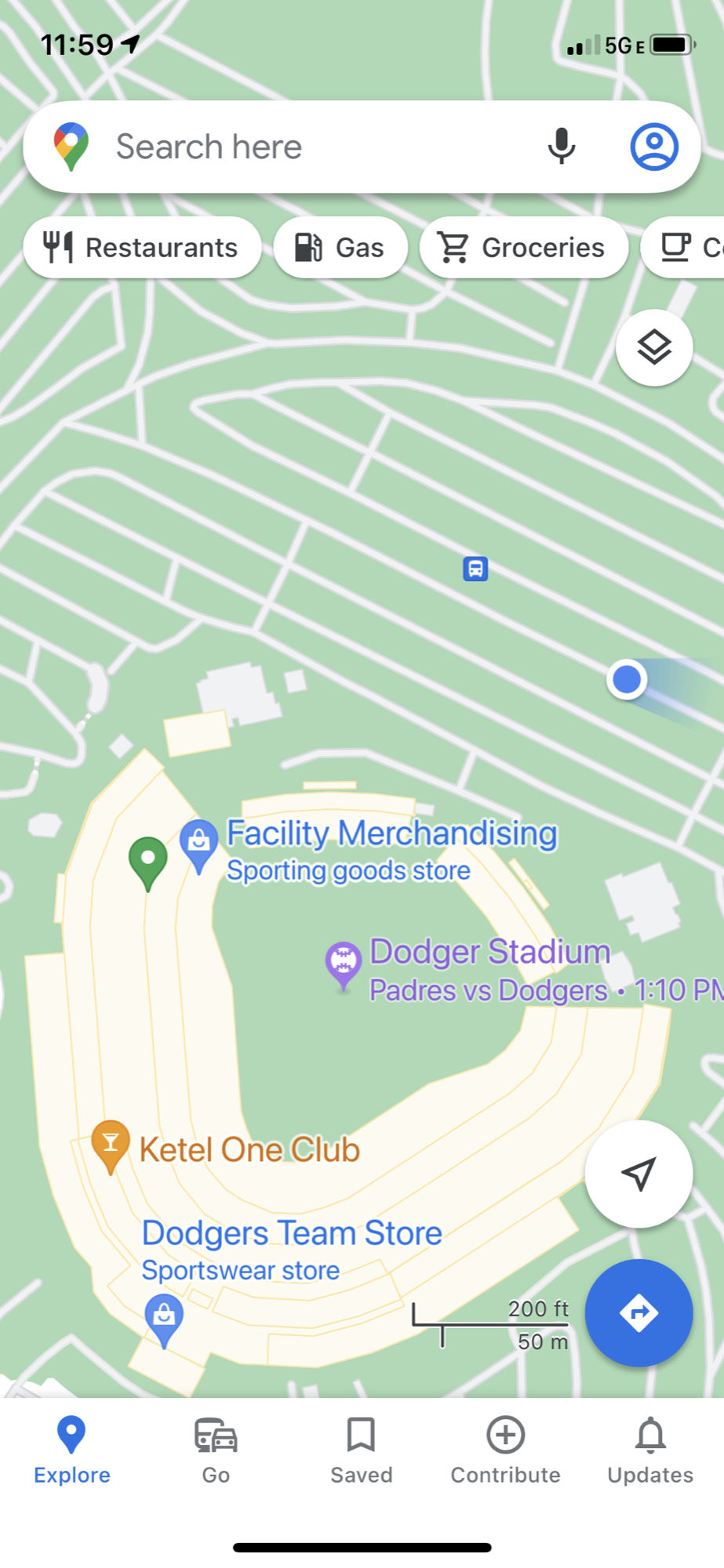A close-up image of a smartphone screen displaying a detailed map of Dodger Stadium. The current time at the top of the screen is 11:59 AM, indicated by a small arrow pointing upwards. The phone has two bars of 5G coverage and a nearly full battery. The Google search bar is prominently featured, complete with a microphone icon and an avatar image. Beneath the search bar, quick access links for restaurants, gas, groceries, and coffee are listed. 

The map highlights the user's location just outside the outfield area of Dodger Stadium, showcasing nearby facilities such as merchandise stores and concession stands. Key points of interest like the Dodgers Team Store and the Ketel One Club are marked. The screen also notes that the Padres are playing the Dodgers at 1:10 PM, suggesting ample time for the user to arrive and explore. Options to navigate, save, contribute, or check updates are available at the bottom of the screen. The overall atmosphere exudes excitement for the game, punctuated by a supportive reminder for Dodgers fans.